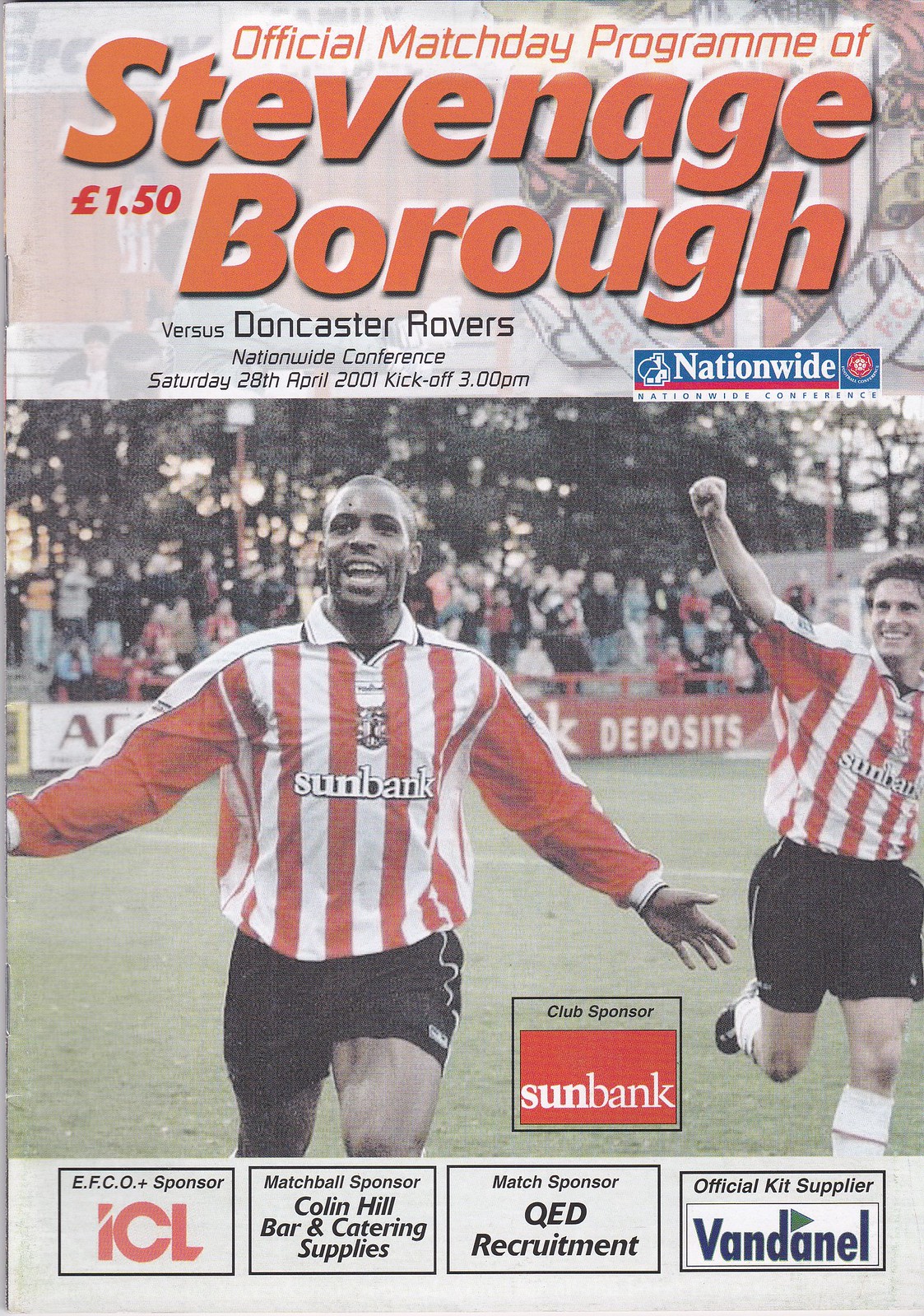The image displays the front cover of the official matchday program for the football match between Stevenage Borough and Doncaster Rovers, held on Saturday, April 28, 2001, with a kickoff at 3 p.m. Sponsored by Nationwide, the event is part of the Nationwide Conference. The program, priced at £1.50, prominently features the emblem of Nationwide, the sponsor.

The cover includes a full-color photograph taken outdoors during the daytime, showcasing a football pitch with a blurred-out crowd and trees in the background under a clear sky. The main image captures two football players from the Sun Bank-sponsored team. The first player, a black male, is in a red and white long-sleeve football shirt and black shorts, with "Sunbank" emblazoned across the chest. The second player, a white male, wears a short-sleeve version of the same red and white shirt with black shorts and is smiling.

Between the players, the club sponsor Sunbank is highlighted in white text on a red background. A white panel at the bottom lists four additional sponsors: EFCO plus sponsor ICL, match ball sponsor Colin Hill Bar & Catering Supplies, match sponsor QED Recruitment, and official kit supplier Vandernal. The photograph gives a sense of the competitive and lively atmosphere of the match day.